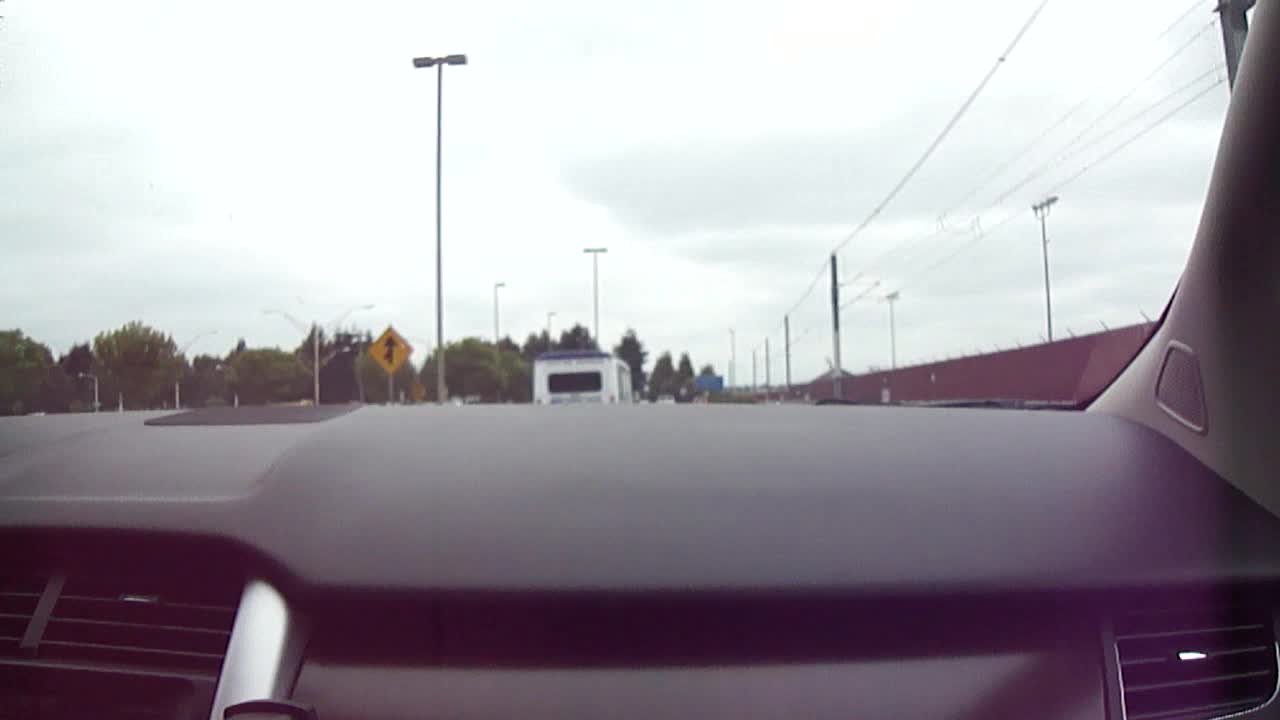This photo, taken from the passenger seat of a car, offers a detailed view of the scene. The bottom third of the image shows the black dashboard with a brownish glove compartment, flanked by two air vents—one on the left and one on the right. Positioned just above the dashboard, the camera captures the road ahead through the windshield. The sky is filled with gray clouds. In the distance, there's a white bus with a blue top directly in front of the car, slightly to the center-right of the frame. On the left, power lines and a series of tall metal poles with lights are visible. Also on the left, a yellow triangular road sign featuring a directional arrow indicates a merging road. A red, very tall chain-link privacy fence runs along the right side of the road. Additionally, there are electrical poles and wires parallel to the road on the right side. The overall atmosphere conveys a typical day of overcast weather on a city road.